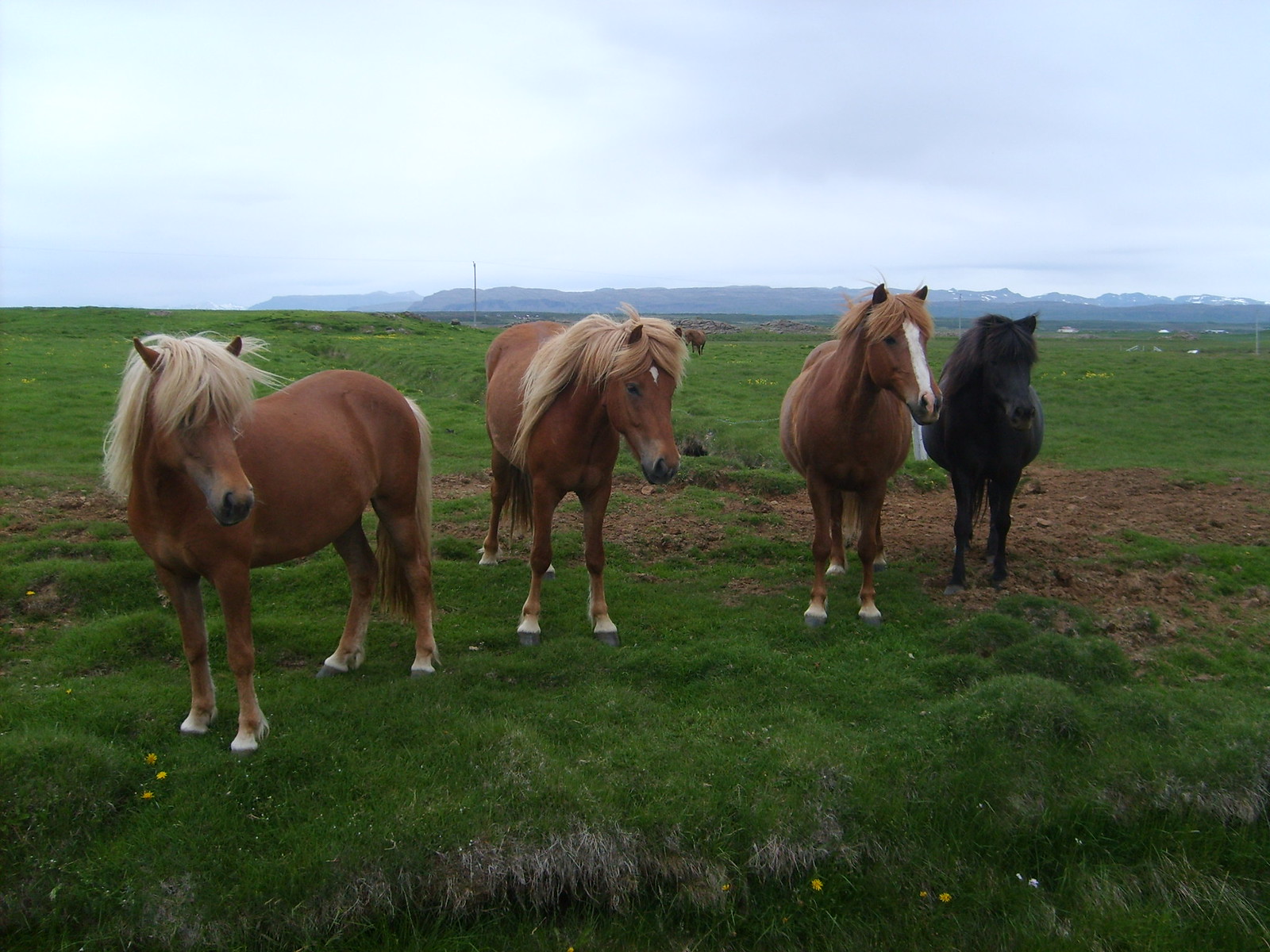The digital photograph captures a lush green meadow on a cloudy day, with an overcast bluish-white sky occupying the upper quarter of the image. The expansive green pasture is dotted with patches of brown grass and a few white and yellow flowers, possibly dandelions. In the foreground, there are four horses grazing. Three of the horses are a warm reddish-brown shade with silky yellow-blonde manes and tails; two of these brown horses have white patches on their faces—one with a spot on its forehead and the other with a stripe running down from its head to its nose. The fourth horse, positioned to the far right, is entirely black. All three brown horses have white hooves, adding to their distinctive markings. Stretching into the horizon are distant, tall hills or mountains in a brownish-green hue, partially blending with the cloud-covered sky.